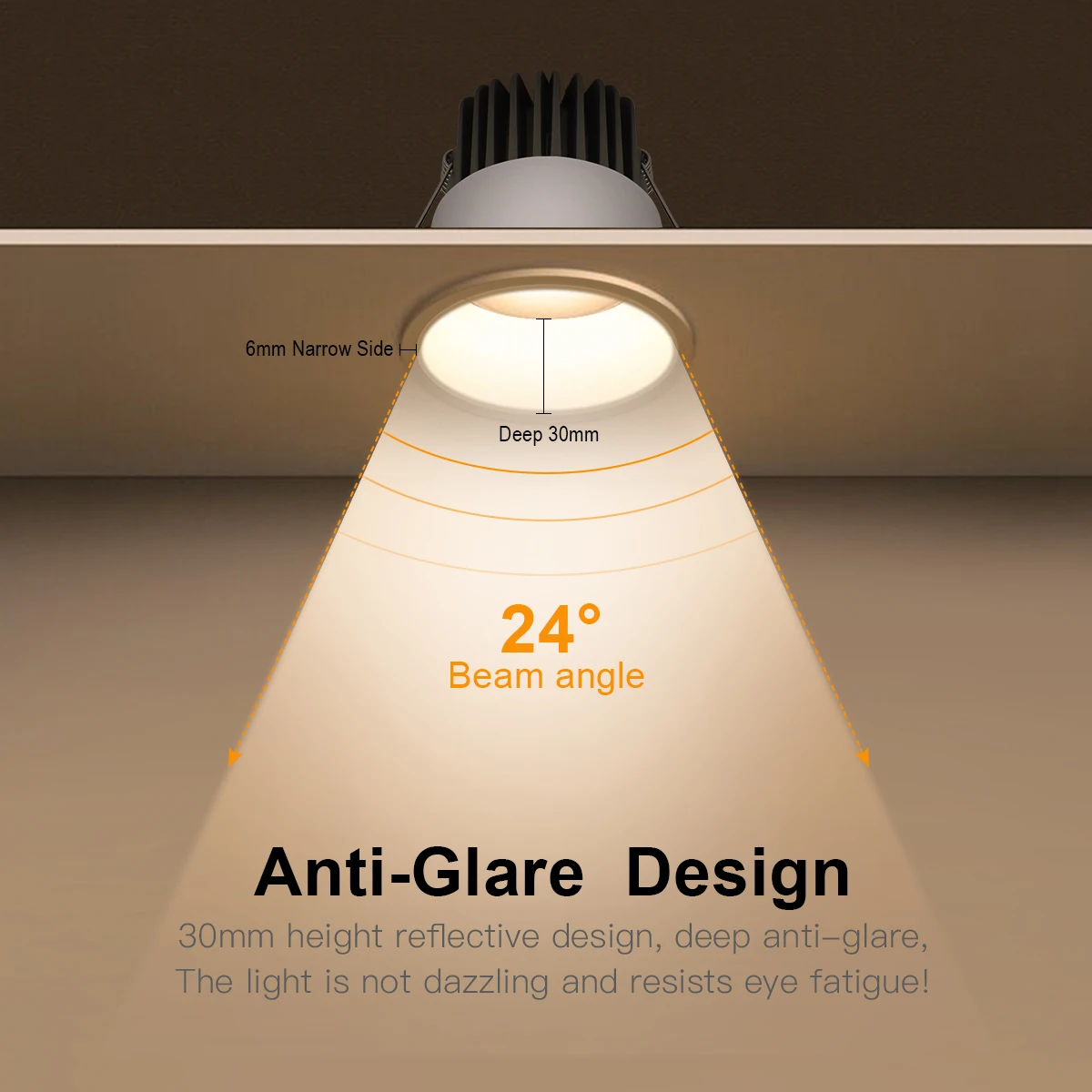This image is a detailed advertisement for a recessed lighting system, possibly a can light. The top section of the image showcases a shelf, representing a ceiling, with a circular opening where the light fixture is installed. From the opening, a cylindrical, steel-like light fixture extends downward, equipped with black fins on top that are partially visible. The fixture casts a triangular beam of light that is wider at the base and narrows upward, indicating a 24-degree beam angle with an anti-glare design to minimize eye fatigue.

Text annotations describe the product's specifics: 
- To the left of the fixture in black font, it mentions "6 millimeters narrow side."
- Below this, also in black font, "deep 30 millimeters."
- Within the triangular light beam, text in orange reads "24° beam angle."
- Below the orange text is more black font stating "anti-glare design."

Further descriptive text below this reads:
- "30 millimeters height, reflective design,"
- And reiterates the feature: "Deep anti-glare. The light is not dazzling and resists eye fatigue."

The overall tone communicates the detailed structure and benefits of the light fixture, emphasizing its design to reduce glare and prevent eye strain.